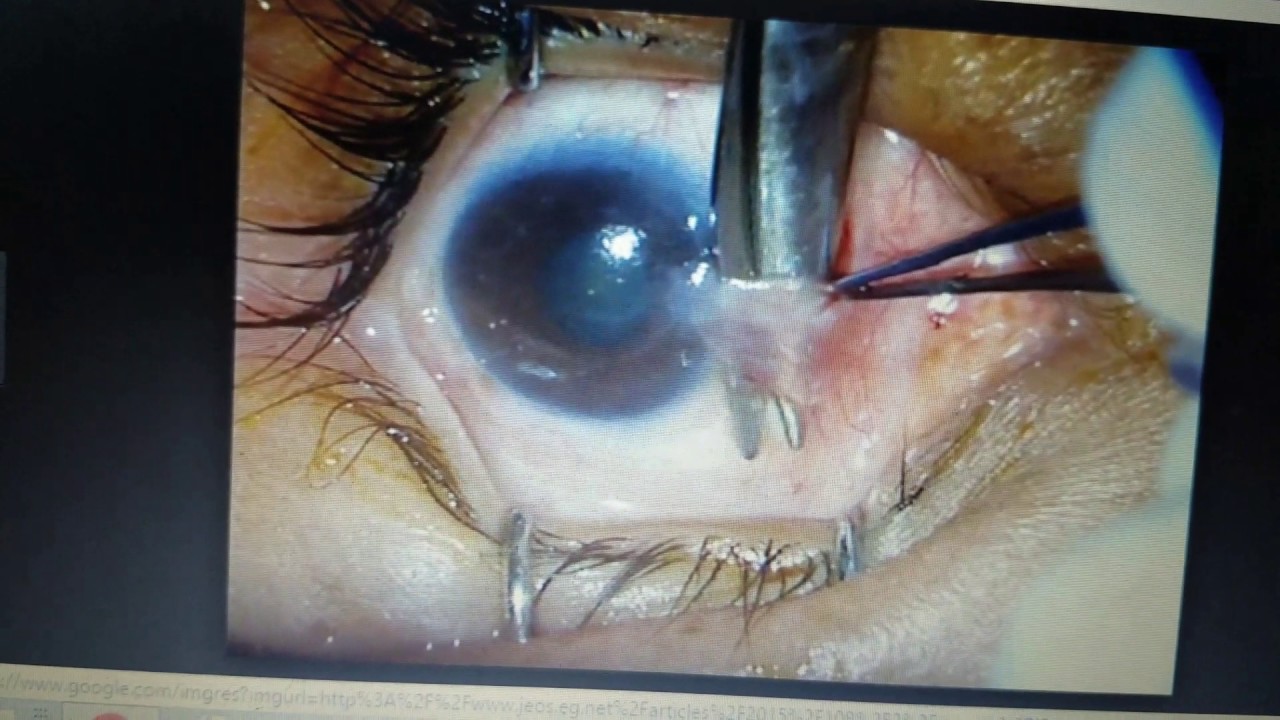The image depicts a detailed and unsettling close-up of a human eye undergoing surgery. The eye is clamped wide open using thin metal hooks, revealing its cloudy sclera with a hint of visible red blood vessels. The upper and lower eyelashes are wet and pushed aside. A pair of metal tweezers, operated by a gloved hand, are peeling back part of the sclera, exposing the inner layers of the eye. A sharp, scissor-like instrument is puncturing the eye, cutting through the sclera with precision. The surrounding skin around the eye is slightly wrinkled and shows a mix of lighter and darker tones, including areas that appear almost brown. The image has a black border, and a link to the Google website is visible at the bottom, suggesting it might be a screenshot from a computer screen. The overall scene is quite unnerving, evoking discomfort due to the invasive nature of the procedure.